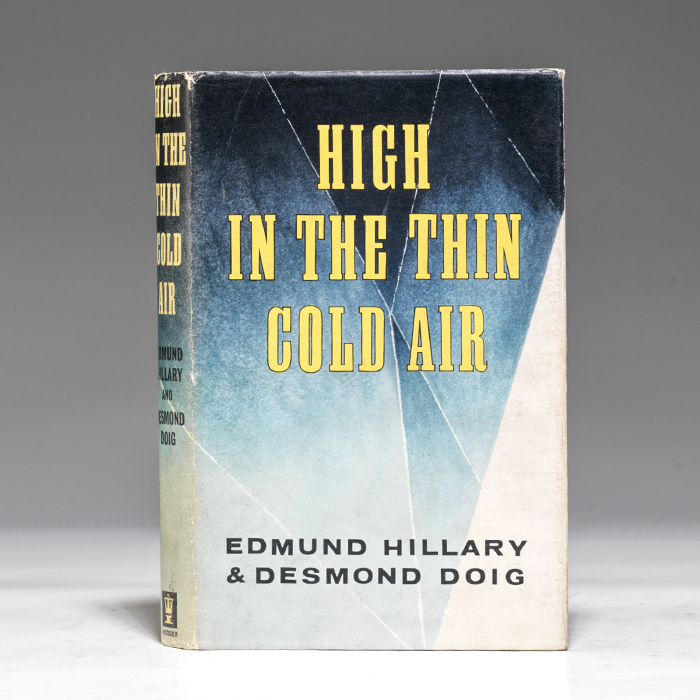The image features a detailed view of the front cover and a portion of the spine of a paperback book titled "High in the Thin Cold Air" by Edmund Hillary and Desmond Doig. The book is positioned upright on a surface that mimics marble, though the exact setting is unclear due to the photograph's emphasis on the book itself. The background is a plain, soft grey, subtly darker at the top, creating a neutral backdrop that highlights the book.

The cover of the book is designed with an abstract, rhombus-shaped gradient pattern. It transitions from a deep blue at the upper section to a lighter blue towards the bottom, finally merging into white. Intricate lines reminiscent of diamond cuts run through this gradient, enhancing the geometric aesthetic.

The title, "High in the Thin Cold Air," is prominently displayed in bright yellow text at the top of the cover, while the authors' names, Edmund Hillary and Desmond Doig, are printed in black text at the bottom. The spine of the book mirrors this design, featuring the same title in yellow and the author's names in black, alongside the publisher's logo resembling a Greek-style fountain at the base.